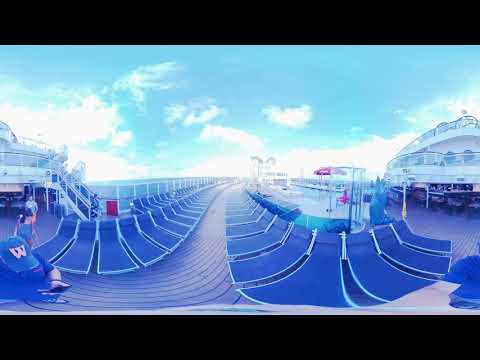The image captures a vibrant scene on the deck of a cruise ship under a bright blue sky dotted with white clouds. The focal point features an array of blue lounge chairs neatly lined up in a wavy configuration on a wooden deck, each chair accented with white outlines. At the lower left of the image, a person wearing a blue baseball cap with a "W" and a blue t-shirt is engrossed in his phone, while two more individuals walk towards him. To the left, a staircase ascends to an upper deck. Beyond the lounge chairs, glimpses of a pool, umbrellas, and different deck levels of the ship are visible, along with a scenic view of the ocean. The sunlight enhances the vibrant colors, capturing the essence of a leisurely daytime atmosphere on the cruise.